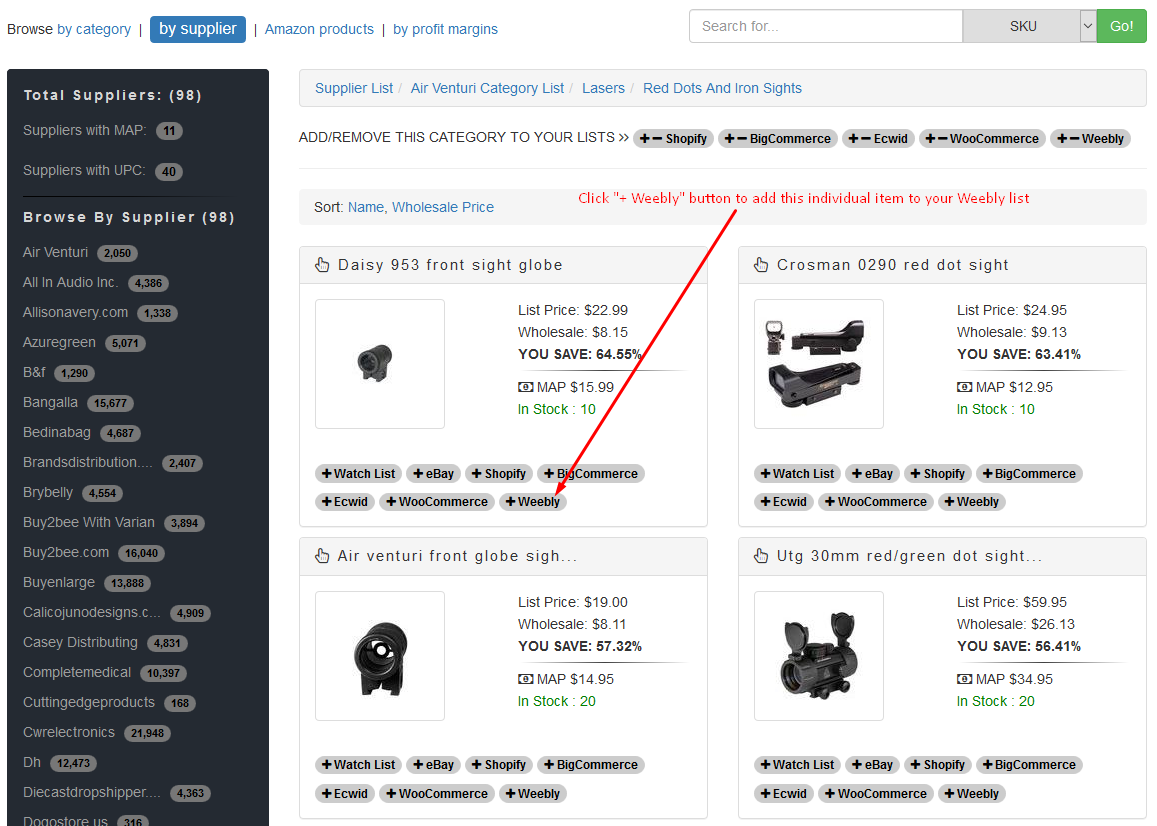Screenshot of the Browse by Category interface on an e-commerce platform, with the "By Supplier" filter selected. The user has navigated to Amazon Products and sorted items based on profit margins. The search bar on the right is set to filter by SKU, with a green "Go" button next to it.

On the left sidebar, under the "By Supplier" filter, the interface displays a breakdown of suppliers: 
- Total Suppliers: 98
- Suppliers with MAP (Minimum Advertised Price): 11
- Suppliers with UPC (Universal Product Code): 40

Below this, a detailed list of suppliers is shown, including:
- Air Venturi: 20 products
- Air Ventan: 2050 products
- All In Audio Inc: 4306 products
- AllisonNavary.com: 1338 products
- Azure Green: 5071 products
- BNT: 1290 products
- Bangalia: 15677 products
- Bed in a Bag: 4687 products
- Brands Distribution: 2407 products
- ...and many more.

The grey bar at the top of the interface is labeled "Supplier List," with a subcategory listed as "Air Venturi Category List: Lasers, Red Dots, and Iron Sights." Beneath this, options to add or remove categories to various shopping carts (Shopify, Big Commerce, ECWID, WooCommerce, and Weebly) are provided. There is also a grey sorting bar which includes options to sort by name and wholesale price.

Highlighted products include:
1. **Daisy 953 Front Sight Globe**
   - List Price: $22.99
   - Wholesale: $8.15
   - Savings: 64.55%
   - MAP: $15.99
   - In Stock: 1 unit
   - Options: Watchlist, eBay, Shopify, Big Commerce, ECWID, WooCommerce, and Weebly
   - A red click-to-add button for Weebly is shown, indicated by a red arrow under this product.

2. **Crossman 0290 Red Dot Sight**
   - List Price: $24.95
   - Wholesale: $9.13
   - Savings: 63.41%
   - MAP: $12.95
   - In Stock: 10 units
   - Options: Watchlist, eBay, Shopify, Big Commerce, ECWID, WooCommerce, and Weebly

3. **Air Venturi Front Globe Sight**
   - List Price: $19.00
   - Wholesale: $8.11
   - Savings: 57.32%
   - MAP: $14.95
   - In Stock: 20 units
   - Options: Watchlist, eBay, Shopify, Big Commerce, ECWID, WooCommerce, and Weebly

4. **UTG 30mm Red/Green Dot Sight**
   - List Price: $59.95
   - Wholesale: $26.13
   - Savings: 56.41%
   - MAP: $34.95
   - In Stock: 20 units
   - Options: Watchlist, eBay, Shopify, Big Commerce, ECWID, WooCommerce, and Weebly

Each product is accompanied by an image located in the left-hand corner of their respective boxes. The interface provides a comprehensive view of product details, stock availability, and various options for integrating with different e-commerce platforms.